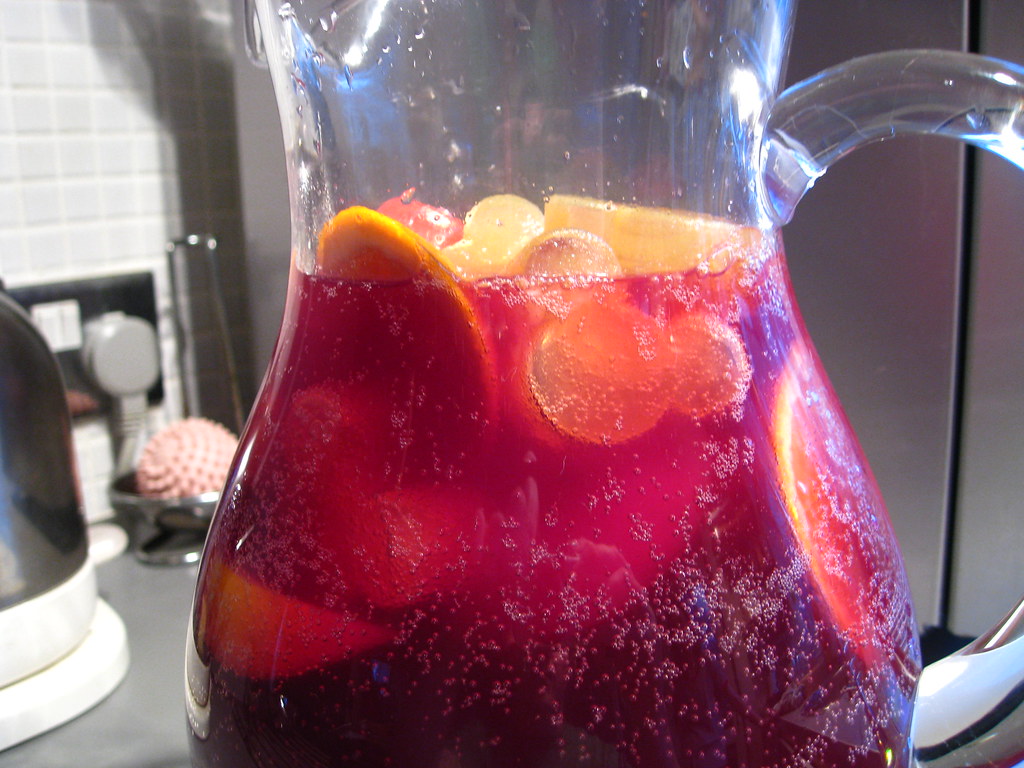In the image, a glass pitcher of red sangria filled with vibrant, sliced citric fruits and bubbling with carbonation sits on a gray kitchen counter. The pitcher, which has a handle, is positioned in a modern kitchen featuring a predominantly gray and white color scheme. To the left of the pitcher, some kitchen appliances are partially visible, including a black kettle on a white base and a gray plug plugged into a silver outlet. A rack is present in the background, along with a distinctive pink laundry ball with spikes in a silver holder. The wall behind the pitcher boasts a gray and white tiled backsplash. Sunlight streams through a window on the right side, casting a reflective glow on the glass pitcher and contributing to the overall bright ambiance of the scene.